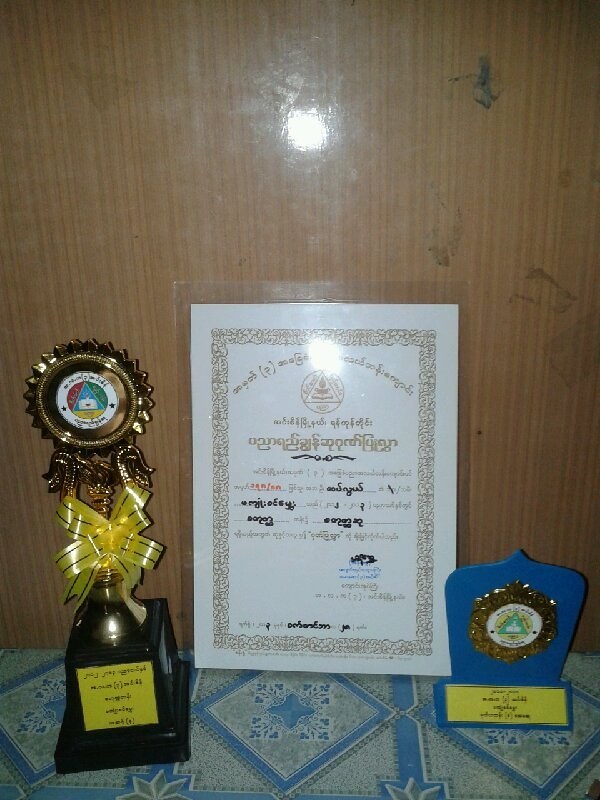This is a detailed photograph taken indoors, showcasing a central laminated certificate that appears official, possibly an award written in a foreign language and potentially reversed due to a reflection. The certificate, off-white in color and rectangular in shape, contains some filled-out sections likely including dates and signatures. To the left of the certificate stands a trophy featuring a circular design with an added yellow ribbon and a card on the front bearing unreadable text, set on a dark stand. On the right side of the image is a smaller, square-shaped blue trophy accented with yellow and containing a central gold circle with white details. All three items rest on a textured blue and white tablecloth patterned with diamonds and floral designs, with a backdrop of brown wood paneling. The scene is highlighted by a flash, contributing to some reflections and partial obstructions in the photograph.